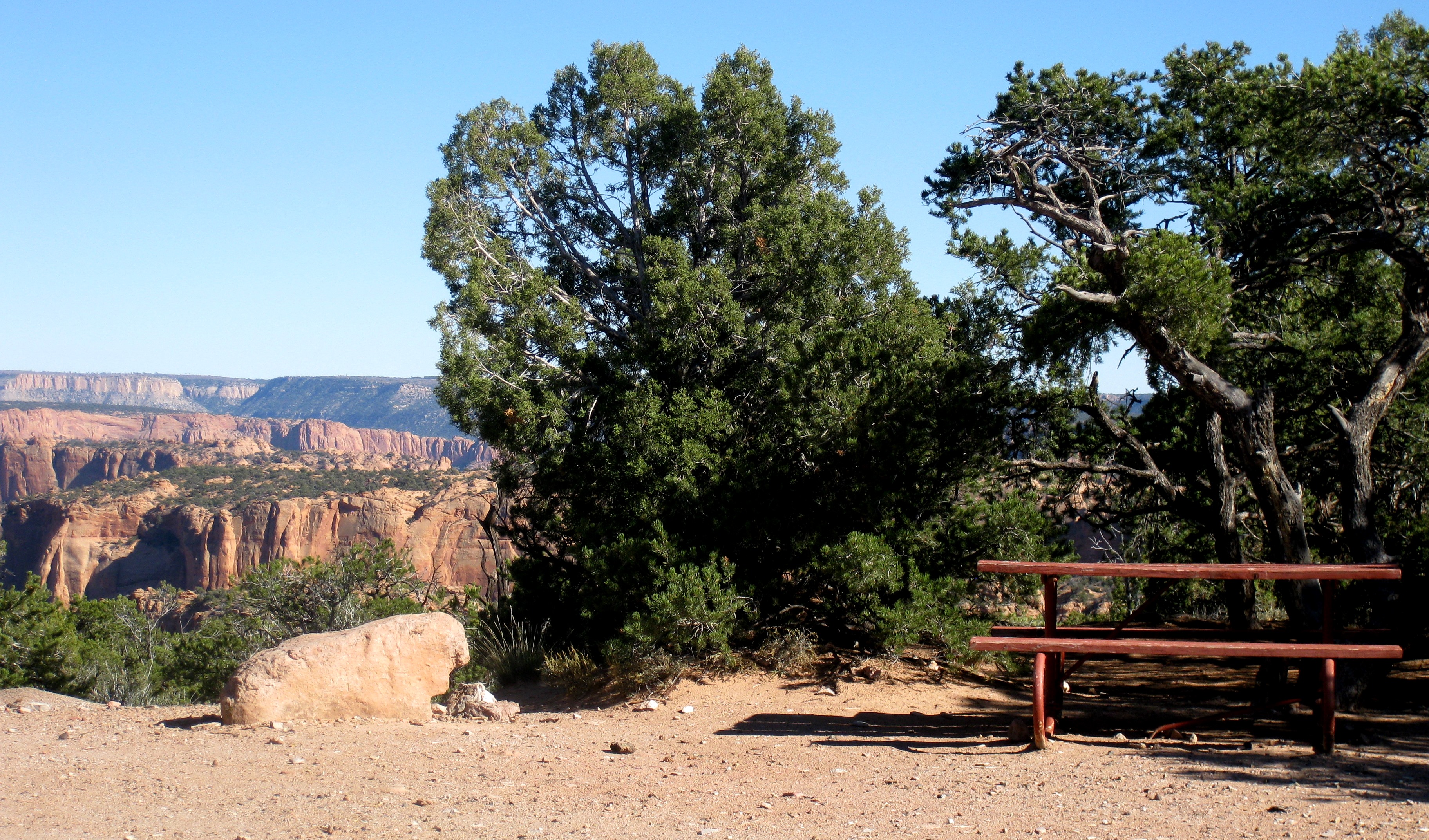The landscape photo showcases a stunning canyon view under a pure, cloudless, Carolina blue sky on a bright sunny day. The canyons are positioned to the left, displaying striking brown rock formations interspersed with patches of green bushes. In the foreground on the lower right, a wooden picnic bench sits atop a sandy and rocky ground, casting distinct shadows, indicative of the sun's position to the right. Scattered white rocks and a prominent boulder add texture to the sandy terrain. Surrounding the scene are tall, bushy green trees with dark brown trunks and thick foliage, some of which cover the middle ground of the photo. This scenic overlook offers an expansive view of the distant mountains and greenery below, possibly capturing the essence of a national park like the Grand Canyon.